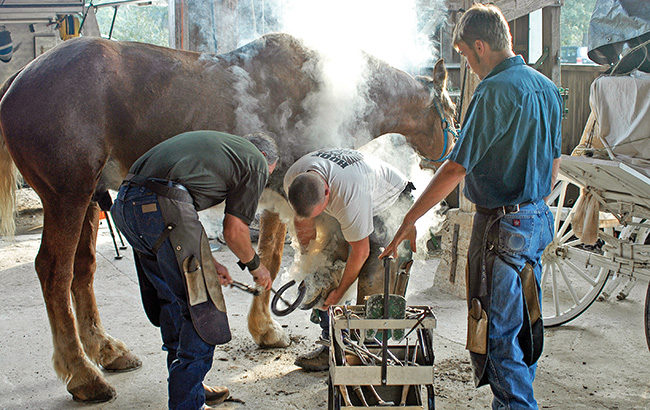In this detailed image, three men are actively engaged in the intricate process of shoeing a horse. Each man is clad in jeans, t-shirts, and protective aprons to guard against the heat and dirt. To the right, one man is observing while the others work. The man in the center, wearing a white shirt, has the horse's hoof lifted, clearly preparing it for the horseshoe. The third man on the left is fitting the horseshoe onto the hoof. The scene is enveloped in steam and smoke, likely emanating from the heated tools and the horseshoe. The horse, a large brown creature, stands calmly with one foot raised, secured by a halter and appearing undisturbed by the bustle around it. Notably, there is a white cart on the right-hand side, and two long metal rods along with the horseshoe are visible, suggesting the use of specialized equipment. The setting reflects a traditional farrier's workspace, rich in the sounds and smells of ironwork.